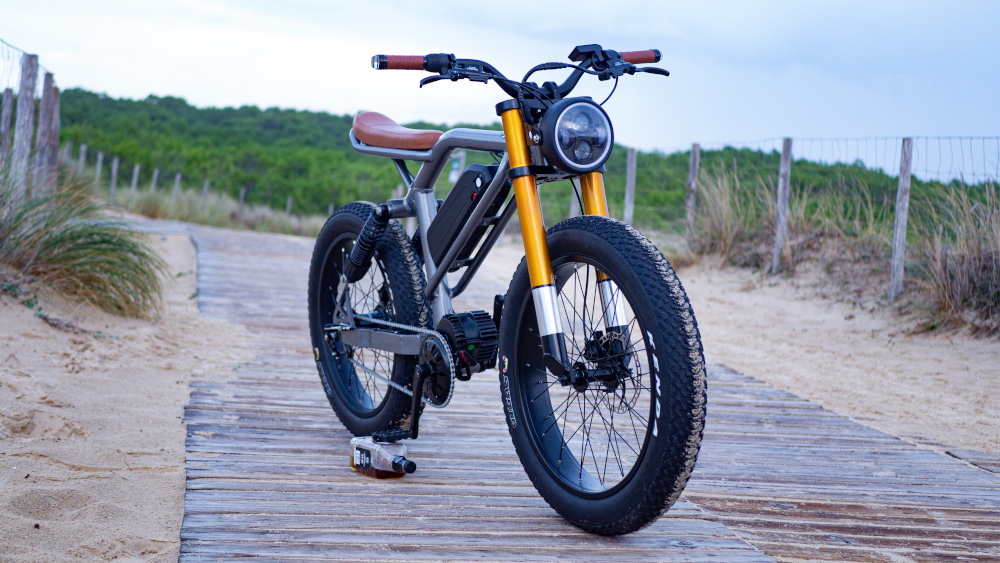In this detailed outdoor photograph, a small mountain bike is prominently featured, parked on a narrow wooden pathway, possibly resembling a boardwalk or a seashore trail. The bike is viewed from the front-right perspective, displaying its distinguishing features. It showcases thick black tires, a brown seat, and handles that are a mix of black and brown. The front portion of the bike is accented with yellow elements, including yellow or gold shocks, and it is equipped with a spotlight.

An electric motor is attached between the pedals, with the battery positioned underneath the seat, indicating that it's a motorized mountain bike. A notable detail in the photo is the Jack Daniels liquor bottle placed beneath the bike's frame, supporting it on the wooden pathway.

The surrounding environment includes some dried weeds and patches of green grass flanking the sides of the path, framed by low fences. In the background, a mix of green trees and sparsely vegetated hills are visible under a blue sky with overcast conditions, suggesting a bright but diffuse sunlight typical of midday. The scene hints at a location near a sandy beach or sand dunes, contributing to the rustic, coastal atmosphere of the photograph.